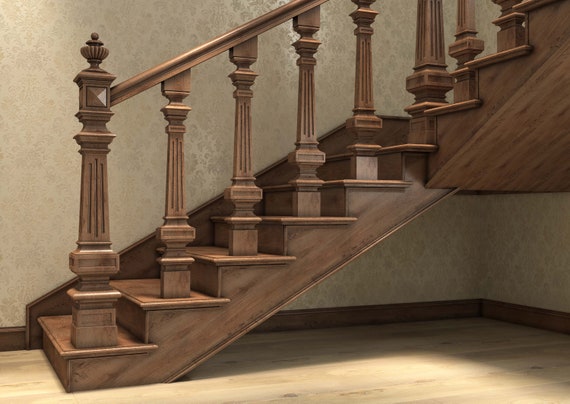The photograph captures an intricately designed wooden staircase situated in what appears to be a residential room. The staircase, composed of luxurious walnut-shaded wood, showcases a detailed handrail supported by finely carved balusters reminiscent of Greek or Doric columns. These decorative balusters feature square tops that taper down, adding elegance to the overall structure. The staircase ascends eight steps before turning at a landing and then continues upward, a feature clearly visible in the image. The light brown hardwood flooring beneath complements the darker, rich tones of the staircase, while a dark brown painted molding delineates the base of the floor. The background highlights a beige wallpaper with a subtle floral pattern, adding to the room's refined ambiance. The right-hand side of the image shows the room's corner, further emphasizing the staircase's central placement. Additionally, there is a small storage space underneath the stairs, suggesting practical use. Overall, this image emphasizes the staircase's craftsmanship and its harmonious integration into the elegantly designed room.